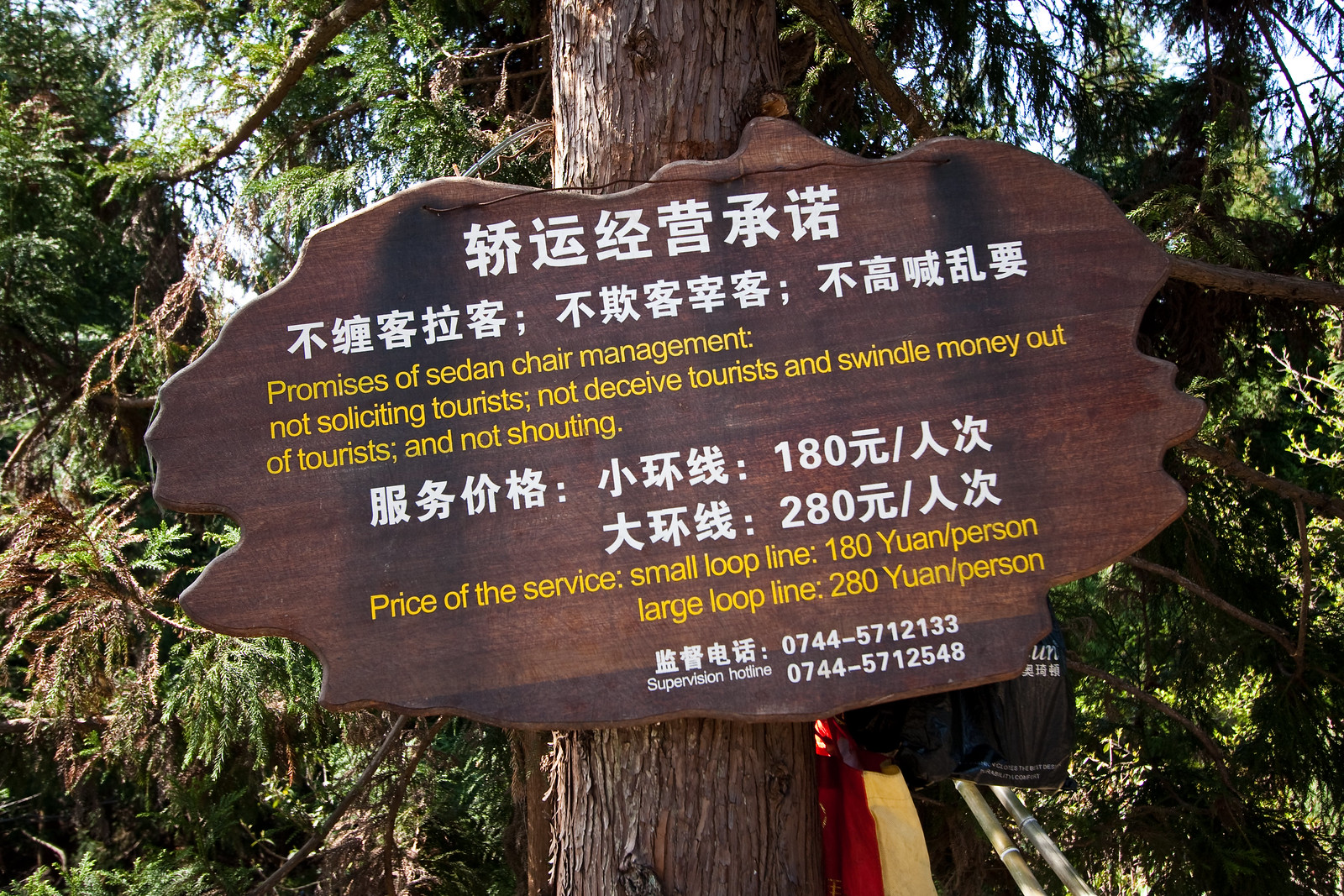This full-color daytime photograph captures a natural outdoor setting in the woods, highlighting a pine tree prominently at the front center. Affixed to the tree is an irregularly shaped wooden sign with both Chinese and English text, each in distinct colors—white for the Chinese characters and yellow for the English translations. The sign is titled "Promises of Sedan Chair Management" and lists rules such as "Not Soliciting Tourists," "Not Deceive Tourists and Swindle Money Out of Tourists," and "Not Shouting." Further down, it outlines service prices: "Small Loop Line 180 Yuan Per Person" and "Large Loop Line 280 Yuan Per Person," accompanied by phone numbers. The background teems with branches and leaves, bathed in sunlight, enhancing the lush, wooded atmosphere. On the right side of the image, a black plastic bag protrudes from behind the sign, and at the bottom, near the tree trunk, there is an unidentifiable red and yellow object.